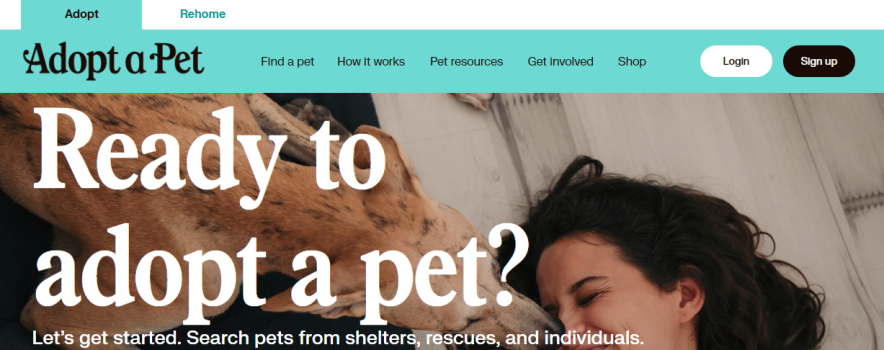The image depicts a webpage with an open tab titled "Adopt," highlighted in bold font. Next to it, a teal-colored tab labeled "Rehome" is positioned. Under the "Adopt" tab, several smaller options are listed: "Find a Pet," "How it Works," "Pet Rescue," "Get Involved," and "Shop." On the top right corner, there are two buttons: a white "Log In" button and a black "Sign Up" button. Below, the page features a prominent header that reads, "Ready to adopt a pet? Let's get started. Search pets from shelters, rescues, and individuals." Beneath this header, there's an image of a woman with brown hair, her face crinkled up in delight as a dog licks her cheek. The dog, difficult to identify clearly due to overlaying text, appears to have a light tan coat, suggesting it might be a golden retriever or a labrador.